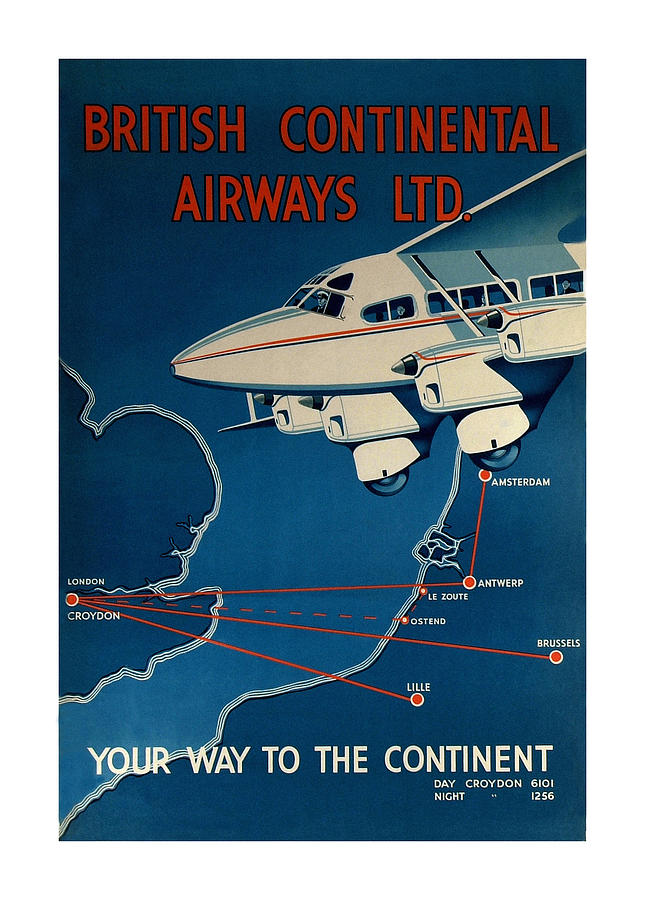The advertisement is an illustrated promotion for British Continental Airways Limited, featuring a vibrant and colorful style suggestive of a vintage era. Dominating the top of the image is the airline’s name, "British Continental Airways Limited," boldly inscribed in red lettering against a dark blue background. Below this, a white jet plane with light blue accents and red and white stripes is depicted flying from right to left. The plane's windows reveal animated passengers and even the pilot, and its landing gear is visible.

Underneath the plane, a map is presented with dark blue landmasses and lighter blue oceans. This map highlights various destinations connected by the airline, such as London, Croydon, Amsterdam, Antwerp, Brussels, and Lille. Red circles mark the important locations, and lines extend from London, showing the routes available. At the bottom of the illustration, in white text, the tagline “Your way to the continent” is prominently displayed, emphasizing the airline's connectivity to continental destinations.

Towards the bottom right, contact information is provided, listing “Day Croydon 6101, Night 1256,” which adds a touch of authenticity and historical context to the overall advertisement.